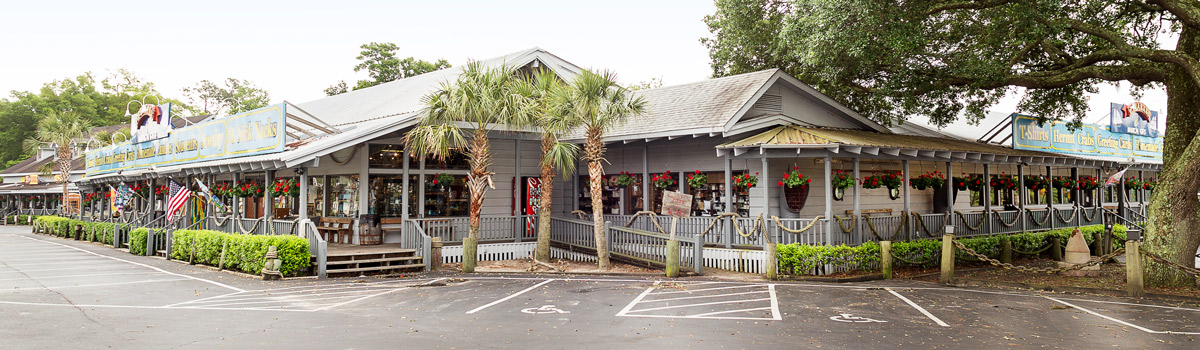In this image, the focus is on a large building, possibly a restaurant, situated in the center. The building, which has the appearance of a sizable house but is too large to be one, is painted entirely in gray with an awning surrounding it. One part of the awning has a yellow roof, adding a splash of color. There are American flags and hanging potted plants with red flowers adorning the exterior. In front of the building, there is a red Coca-Cola vending machine. 

The parking lot, which is blacktop with visible white lines and handicapped parking slots, extends around the building, with no cars currently parked. The lot itself occupies the bottom part of the image. To the right of the building stands a large, curvy tree with green moss and prominent branches extending over the roof. There are also three palm trees at the entryway. On the left and right sides of the image, additional trees and bushes frame the scene. A blue sign and a large green sign with gold text are present, though the text isn't legible. The horizon at the top of the image reveals a light blue sky with some trees, enhancing the setting's warm climate feel. This scene suggests a quiet moment, perhaps captured before the restaurant opens to the public.